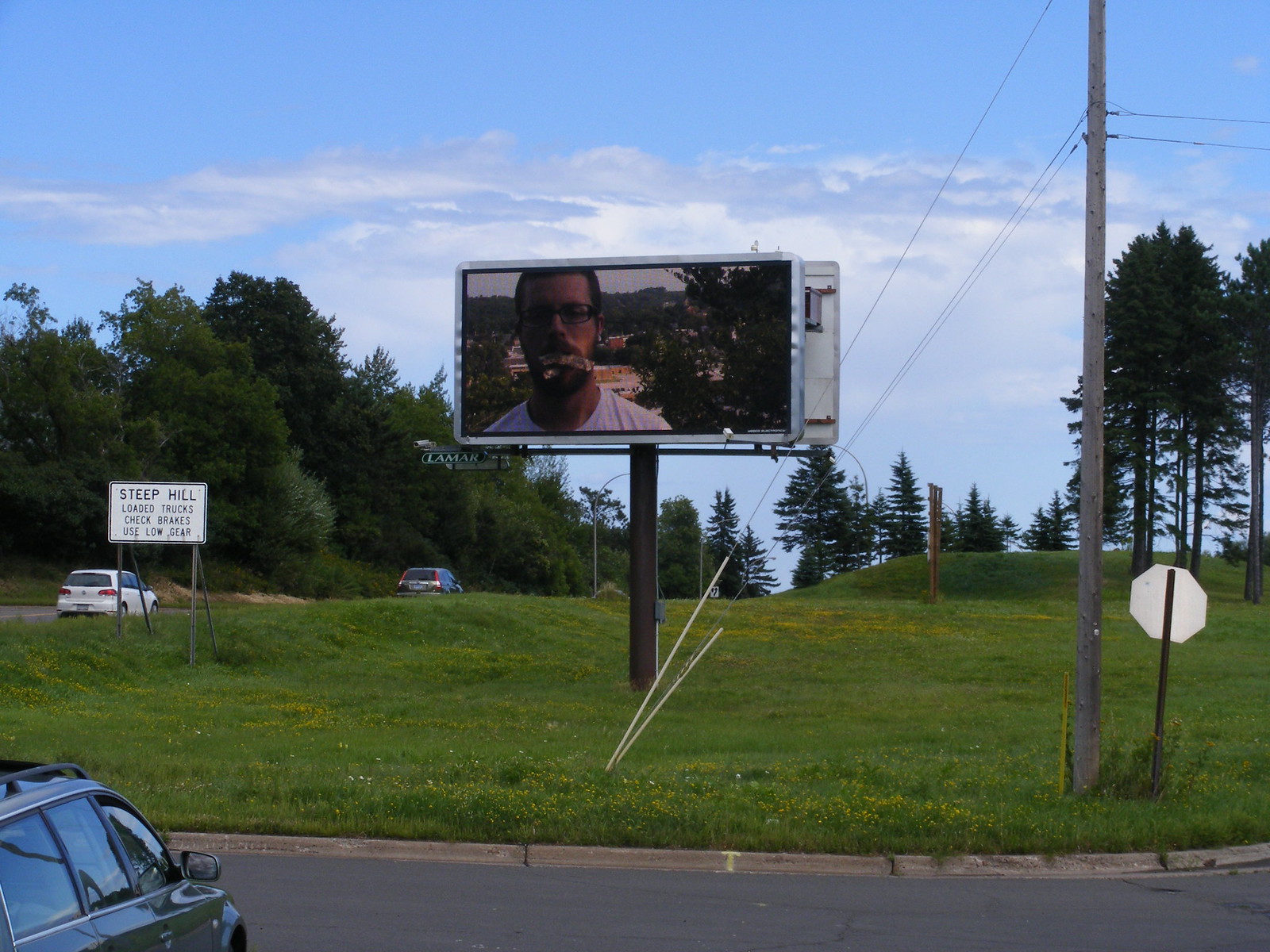The image captures a scene from a parking lot, looking forward at a large expanse of green grass with a prominent billboard in its center. In the bottom left corner, there is a partial view of a green station wagon, showing three side windows and a bit of a roof rack. Adjacent to this, a concrete curb separates the parking lot from the grass area. The grassy field stretches up to about half the height of the image. On the right side of the grass, near the bottom, a power line runs diagonally with three lines attached, and a large pole supporting the billboard is visible. The billboard, which has a gray edge, displays a detailed advertisement featuring a man with short brown hair, glasses, and a white t-shirt. He appears to have something in his mouth. The background of the billboard includes a sky, a mountain range, and a tree on the right side. To the right of the billboard's base, the back side of a silver stop sign is noticeable. A white sign to the left of the grassy area reads "Steep Hill" with additional black lettering detailing road safety instructions for trucks. In the distance, a car can be seen driving away to the right, with another silver car slightly further up. The upper half of the image shows a thick tree line that thins out as it extends rightward, eventually giving way to a blue sky with scattered white clouds. The setting is framed by power lines and additional trees in the background, suggesting an open, suburban area with adjacent roadways.